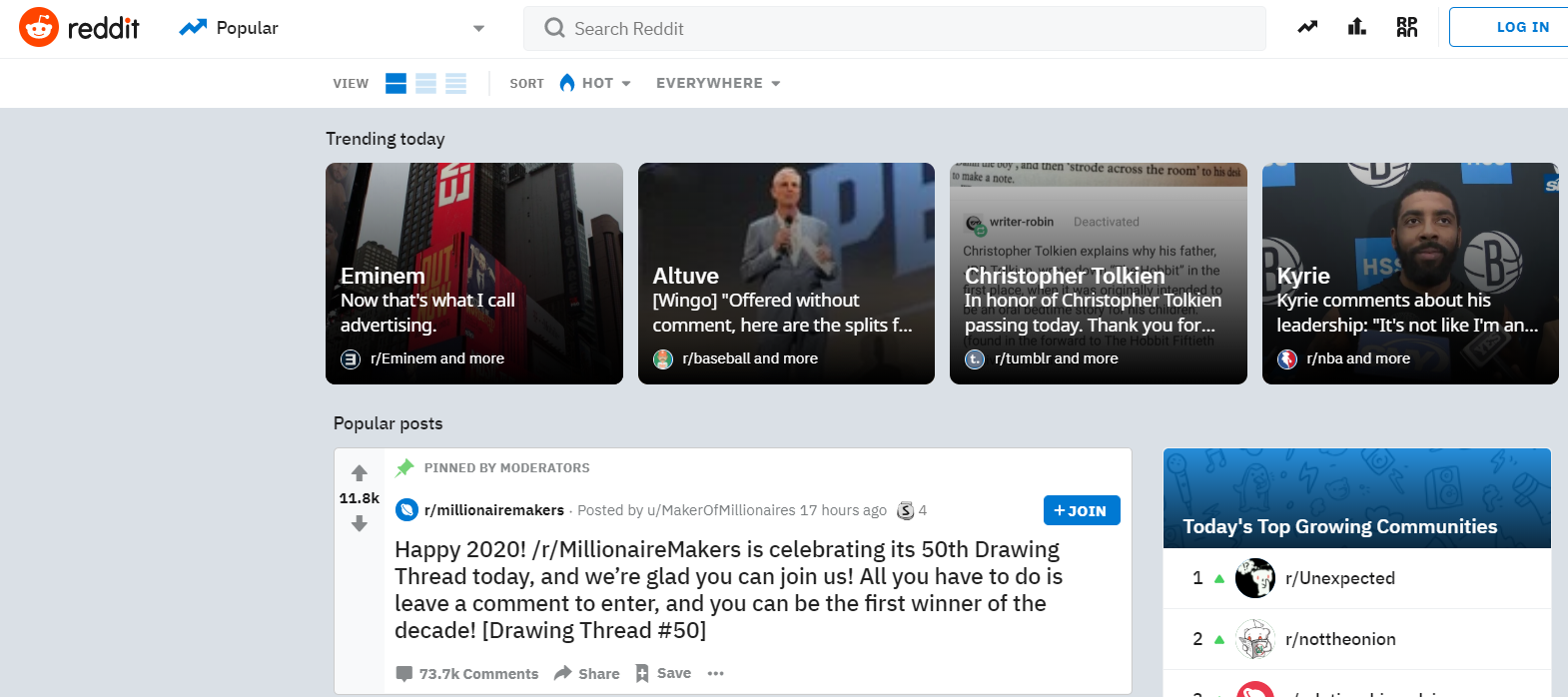This image depicts a Reddit web page from the "Millionaire Makers" community. At the forefront is a comment celebrating the community's 50th drawing thread, wishing a happy 2020 to its members. The comment highlights the excitement of potentially being the first winner of the decade by simply leaving a comment to enter. Notably, the comment mentions the 50th drawing thread in parentheses.

A prominent blue "Join" button, featuring a plus sign, invites users to become members of the community. 

Above this section are four boxes showcasing trending topics for the day: 
1. A visual ad for Eminem with the tagline "Now that's what I call advertising."
2. A post labeled "Out to," offering split information without additional commentary.
3. A tribute to Christopher Tolkien, including an image of a paper, acknowledging his passing.
4. A photo of a man with a headline discussing Kyrie Irving's comments on his leadership, though the text is partially cut off.

At the top of the web page, blue tabs labeled "View," "Sort," "Hot," "Everywhere," and "Popular" provide navigation options for users to explore different threads and content.